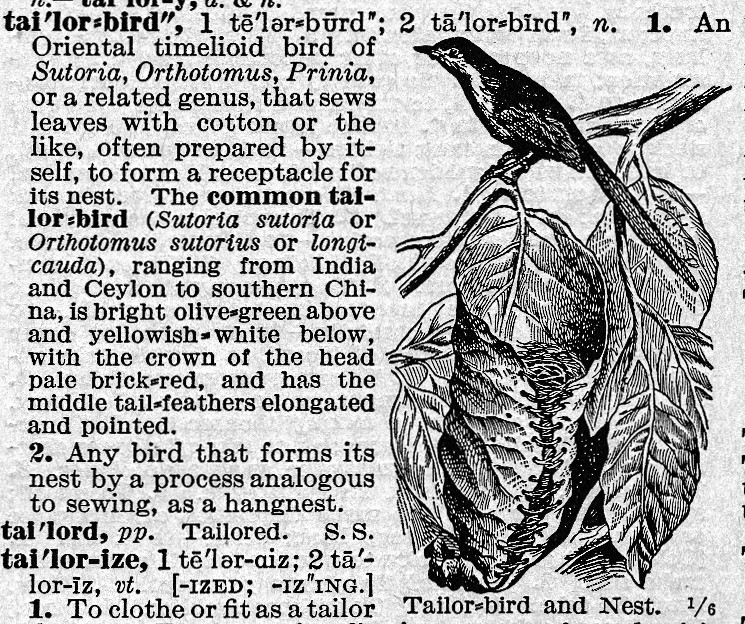The image is a black-and-white excerpt from a dictionary. On the left side, there is text describing the "Taylor Bird," specifically the "common tailor bird" (Sutoria or Orthotomus sutorius). The description provides detailed information about the bird: it is native to regions from India and Ceylon to southern China, with bright olive-green plumage above and yellowish-white below, a pale brick-red crown on its head, and elongated middle tail feathers. The text explains that this bird, or related species, skillfully sews leaves together with cotton or similar materials to create a receptacle for its nest, an activity that gives the bird its name. Below the main entry, there are also entries for "tailored" and "tailorized," defined as "to clothe or fit as a tailor."

To the right of the text, there is an intricate black-and-white illustration showing the tailor bird perched on a branch. The bird is depicted with its tail feathers pointed down and to the right, while it faces to the left. Below the branch, leaves are sewn together to form a cup-shaped nest, emphasizing the bird's nest-building skills that are described in the text. This illustration offers a visual complement to the detailed definitions provided in the textual entries.